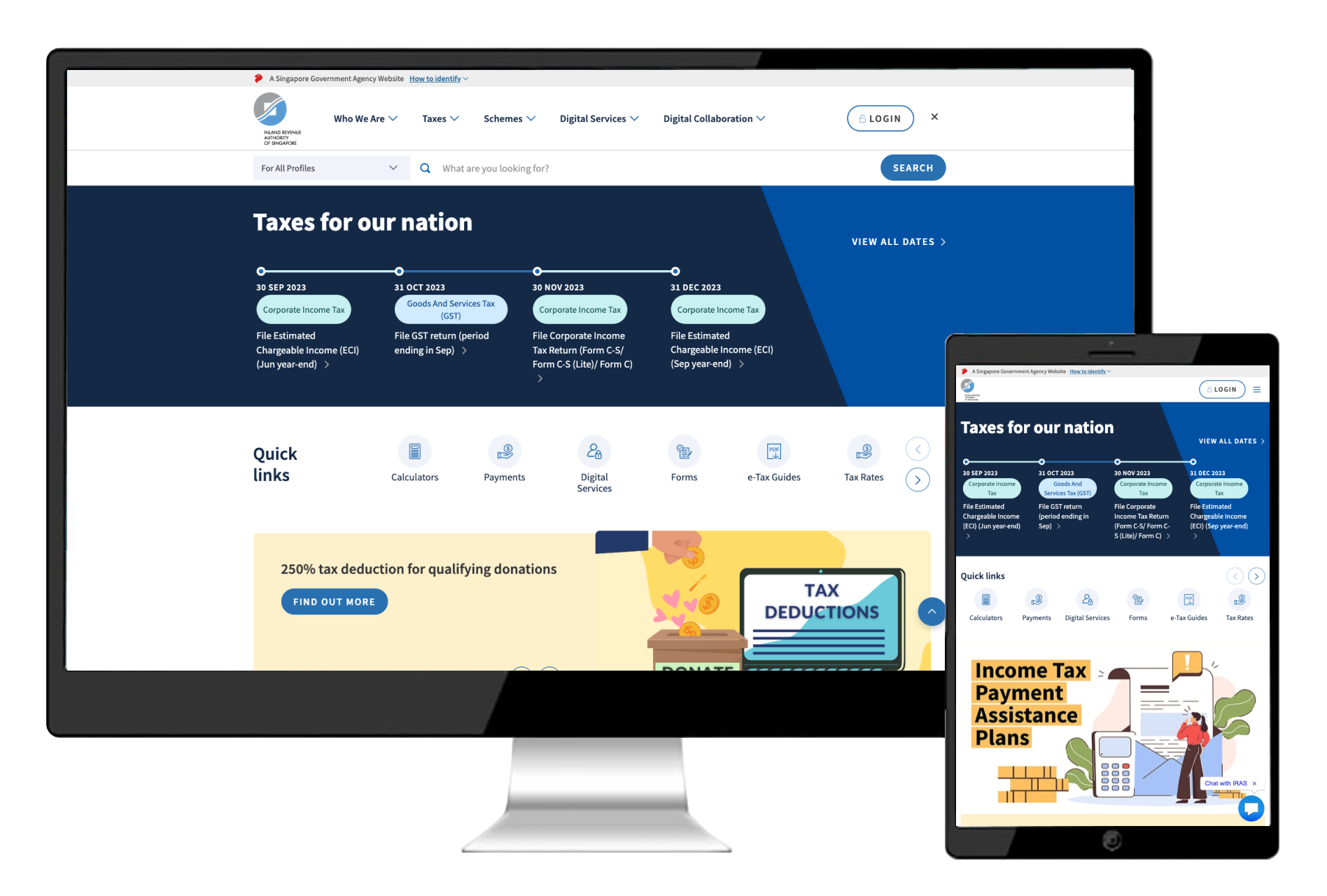A high-resolution image showcases a sleek PC monitor and a tablet side by side. The PC monitor, dominating the left side of the frame, displays a "Taxes For Our Nation" website, featuring a section on tax deductions. Positioned at the front lower right corner of the PC monitor is the tablet, which portrays the same website in its mobile version. The mobile site differs slightly, displaying a banner with the same "Taxes For Our Nation" title and an illustration of a person holding a calculator along with a sheet of paper labeled "Income Tax Payment Assistance Plans." Both devices reflect a modern, digitally connected approach to managing taxes, emphasizing the accessibility of tax-related information across multiple platforms.